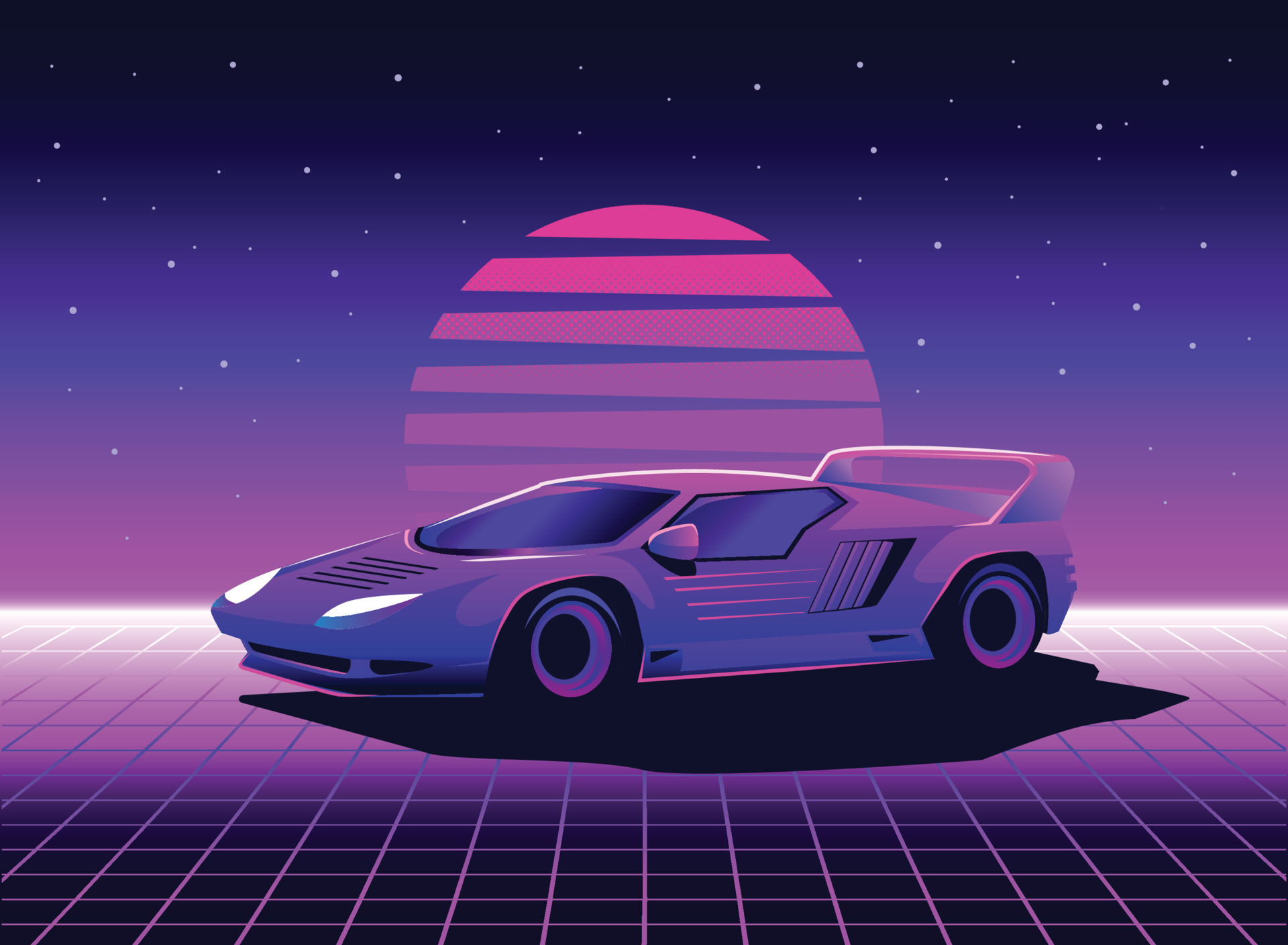A meticulously drawn image features a streamlined, white supercar, embodying the sleek, revved-up aesthetics of an 80s sci-fi futuristic style. The car's small, sporty design is accentuated by its illuminated white headlights and a distinctive carrier rack, which is elevated off the rear. The vehicle is positioned on a grid-like floor comprised of black squares with purple outlines, casting an overall purple hue across the scene. The backdrop showcases a captivating night sky transitioning from dark blue to vibrant pink. Dominating the horizon is a striking, segmented pink moon, flanked by shimmering stars. Below this cosmic arrangement, directly behind the car, a glowing white area enhances the ethereal ambiance of the image.